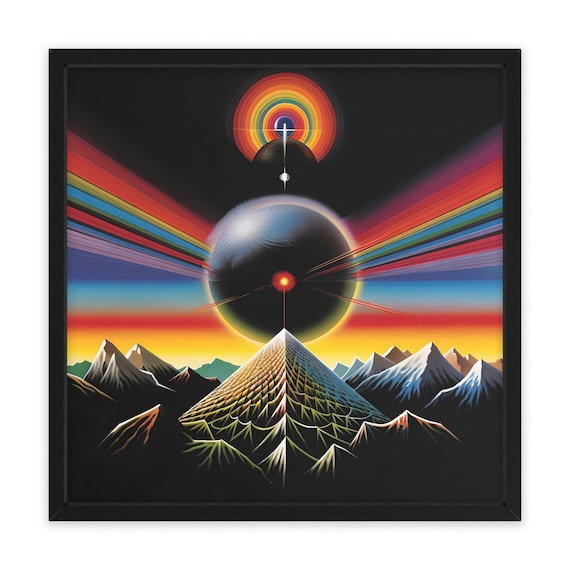The image is a striking visual reminiscent of psychedelic art, much like Pink Floyd's "Dark Side of the Moon" album cover. In the foreground, there are pointed, snow-capped mountain peaks with a prominent pyramid-like formation at the center. This formation leads up to a dark sphere hovering in the sky with a red center dot that emits beams of light in various rainbow colors, spreading across the image. Directly behind this sphere is a slightly smaller black sphere with a white center dot, subtly blending into the dark background. Above these spheres, there is a circular rainbow formation set against an all-black sky. The entire scene is enveloped in a spectrum of vibrant colors – red, orange, blue, purple, and green – creating an ethereal and surreal atmosphere with a retro, psychedelic feel.